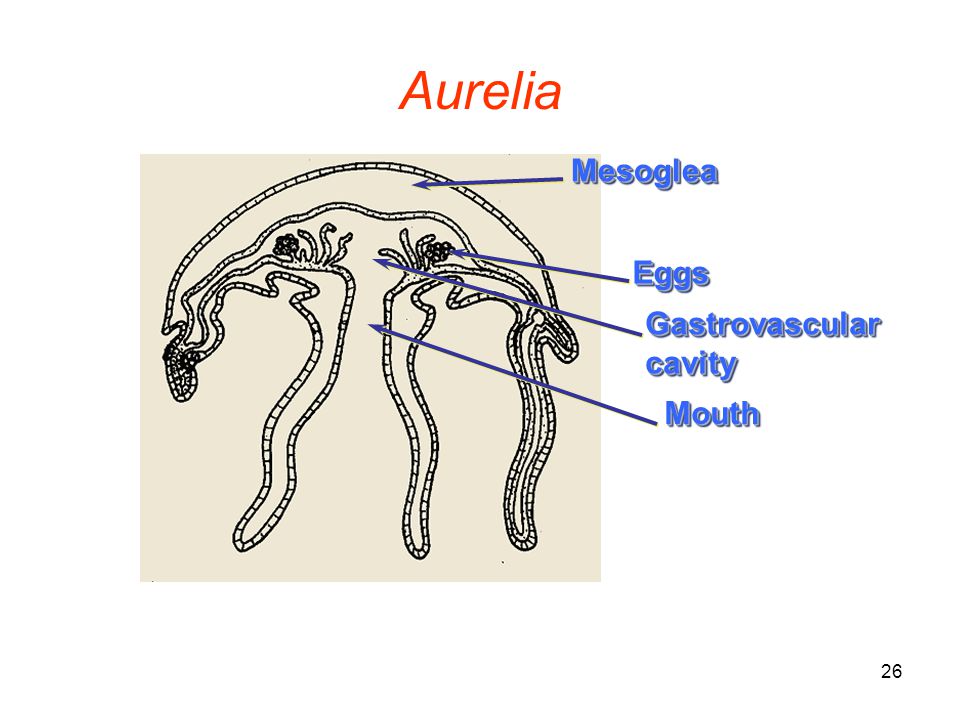The image is a detailed sketch drawing titled "Aurelia" in bold red font at the top. Within a tan-colored square, the black and white drawing depicts a jellyfish-like shape, intricately edged in black and white and segmented into different regions with various internal structures. Along the right-hand side, blue arrows and text labels point to distinct parts of the body. The top dome-like shape is labeled "Mesoglea," beneath which "eggs" are indicated with an arrow. Further below, another arrow marks the "gastrovascular cavity," and finally, an arrow points to the "mouth" at the central opening of the structure. The precise nature of the object depicted remains unclear, possibly suggesting a biological entity such as a jellyfish, virus, or cellular component.